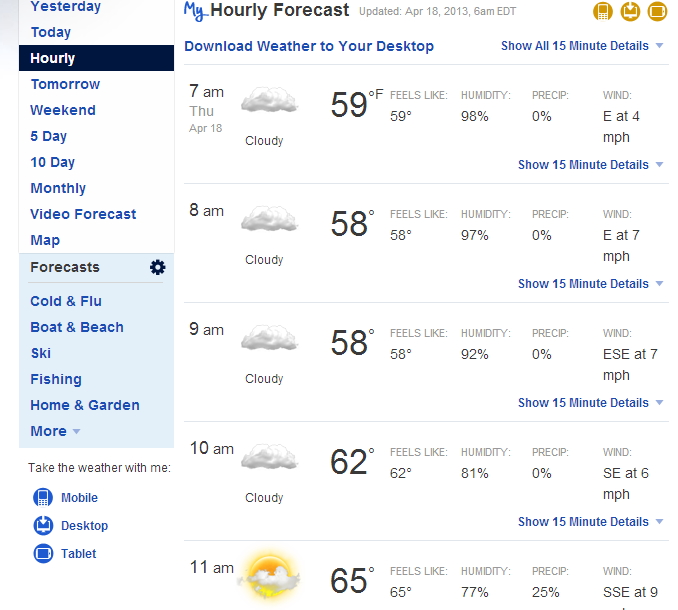A detailed screenshot of the weather application "My Hourly Forecast," captured on April 18, 2013, at 6 a.m., potentially displayed on a variety of devices including an iPad, tablet, desktop, or laptop. The interface features icons representing different screen formats such as phone, computer, and tablet. 

On the left side, a vertical menu lists various sections including Yesterday, Today, Hourly, Tomorrow, Weekend, Five Day, Ten Day, Monthly, Video, Forecast, and Map. Adjacent to this menu, within a bluish box accented by a settings gear icon, a label indicates "Forecasts" with categories tailored to specific interests: Cold and Flu, Boat and Beach, Ski, Fishing, and Home and Garden. These categories provide weather updates relevant to those particular activities.

A prompt to "Download Weather to Your Desktop" is displayed prominently. The center of the screenshot showcases the Hourly Forecast, detailing temperatures ranging from 58°F to 65°F, with significant humidity throughout the morning hours. No precipitation is anticipated until around 11 a.m. The hourly forecast specifies conditions in 15-minute intervals from 7 a.m. through 11 a.m., predicting a mostly cloudy morning with some sunshine peeking through and very mild winds.